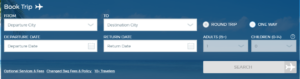The image features a rectangular layout primarily focused on a travel booking interface. In the top left corner, the text "Book Trip" is prominently displayed, followed immediately to the right by a white airplane logo. Below this header, there are four white rectangles arranged in two rows of two, appearing as interactive fields for user input.

To the right of these input fields, two tabs with white text are visible, likely for navigation or categorization purposes. Further down, the image includes two gray rectangles, with a longer light gray rectangle positioned in the bottom right corner. In the bottom left corner, extremely small white text is present, providing additional details or disclaimers. Overall, the image presents a clear and organized user interface for booking travel arrangements.